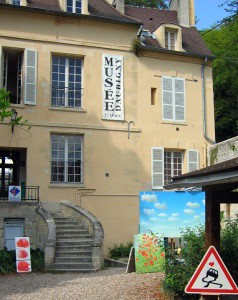This photograph depicts the exterior of what appears to be an old building, possibly a converted residence now functioning as a museum, indicated by a vertical blue flag that reads "MUSEE" in French. The building, made of yellowish-beige stucco, is three stories tall with numerous tall windows and a brown roof. A cement staircase, curving and positioned at an angle, leads up to the first floor. Alongside the staircase are several paintings, seemingly prepared for an exhibit. These include a canvas of red flowers in a field, another of a blue sky with clouds, and a quirky image of a car driving crookedly with a heart above it. A notable detail is a triangular sign at the bottom right, featuring a car slipping, likely a wet road warning. The scene is framed by some trees and a gutter vane, all bathed in sunlight, adding to the vibrant atmosphere of this art gallery setting.